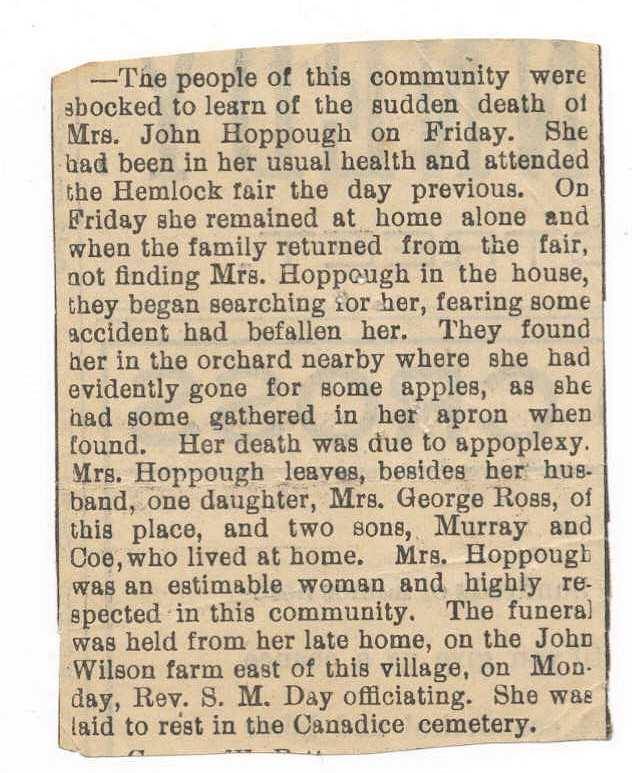This image is a scan of an aged, yellowed newspaper clipping, indicating it is an original and not a photocopy. The clipping is an obituary for Mrs. John Hoppaugh, who passed away suddenly on an unspecified Friday. The community was shocked by her death as she had been in her usual health and had attended the Hemlock Fair the day before. On the day of her passing, she remained at home alone. Upon the family's return from the fair and not finding her at home, they began searching for her, fearing an accident. She was discovered in a nearby orchard with apples gathered in her apron, indicating she had gone to pick apples. Her death was attributed to apoplexy. Mrs. Hoppaugh is survived by her husband, a daughter named Mrs. George Ross, and two sons, Murray and Coe, who lived at home. She was described as an estimable woman, highly respected within the community. The funeral took place at her home on the John Wilson Farm, east of the village, on the following Monday, with Reverend S. M. Day officiating. Mrs. Hoppaugh was interred in the Canadice Cemetery.